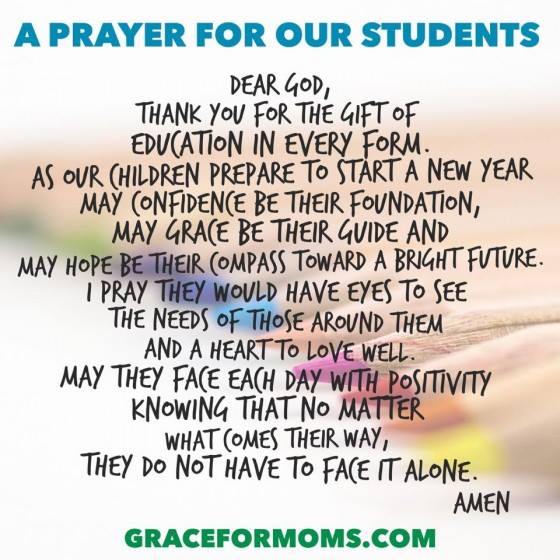This square image features a heartfelt prayer for students, layered over a subtle, somewhat blurred background of various colored pencils against a white backdrop. At the top, in aqua blue text, the heading reads "A Prayer for Our Students." Below, in black text, the prayer begins: "Dear God, thank you for the gift of education in every form. As our children prepare to start a new year, may confidence be their foundation, may grace be their guide, and may hope be their compass towards a bright future. I pray they would have eyes to see the needs of those around them and a heart to love well. May they face each day with positivity, knowing that no matter what comes their way, they do not have to face it alone. Amen." At the bottom, in green text, is the website "Graceformoms.com."